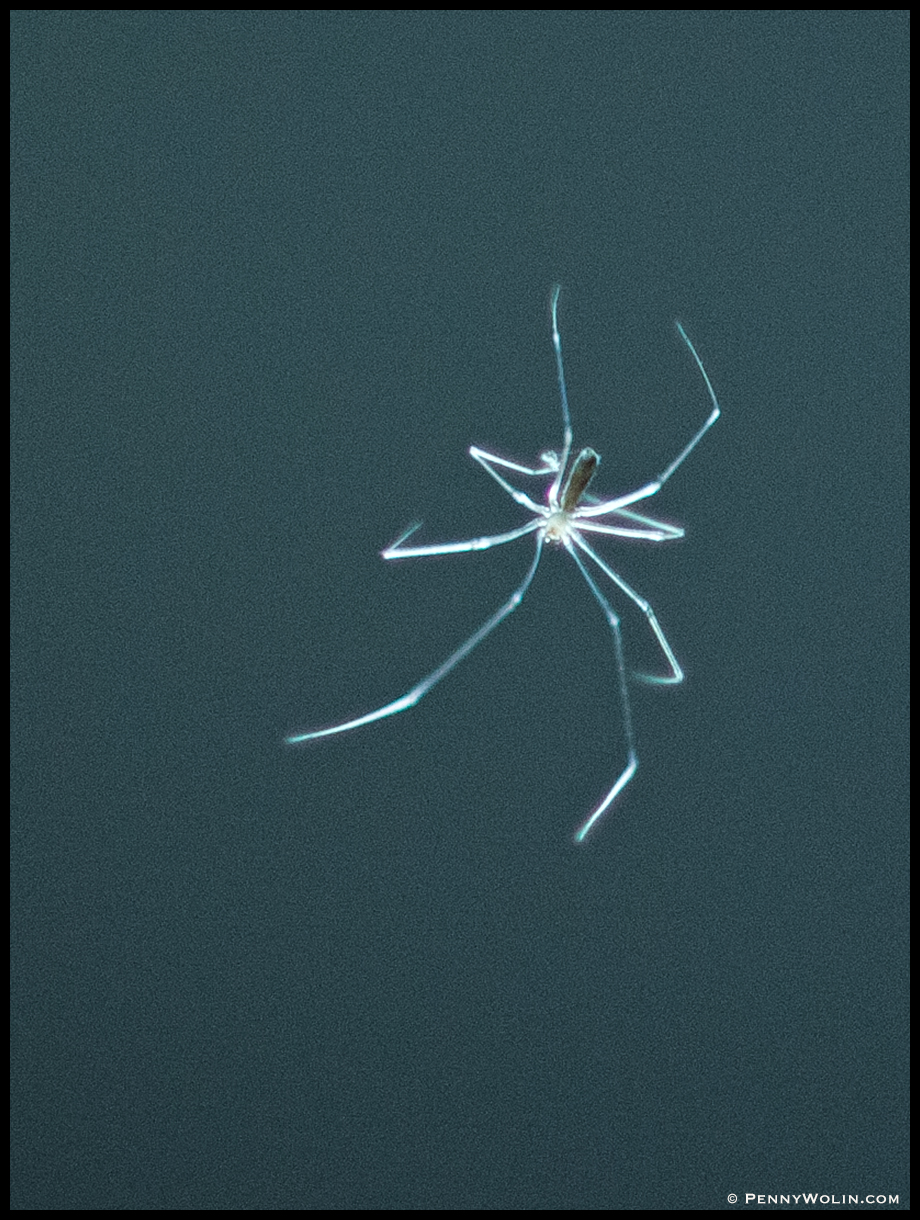This full-color image features a spider set against a dark, nearly black background with an even darker black border. The spider, species unidentified, has extremely long, thin legs similar to those of a daddy long legs, yet they exhibit a slightly translucent, ghostly white appearance with red highlights where the light strikes. The backdrop appears to be a gray-blue, suggesting an underwater setting, although this is not definitively confirmed. The spider's body includes a small, nearly indistinguishable head and a larger, grain-of-rice-shaped abdomen. Despite being an arachnid, the photograph might create the impression of it having six legs due to the angle or positioning. In the bottom right corner, white text reads "pennywolin.com," indicating the photographer's website.